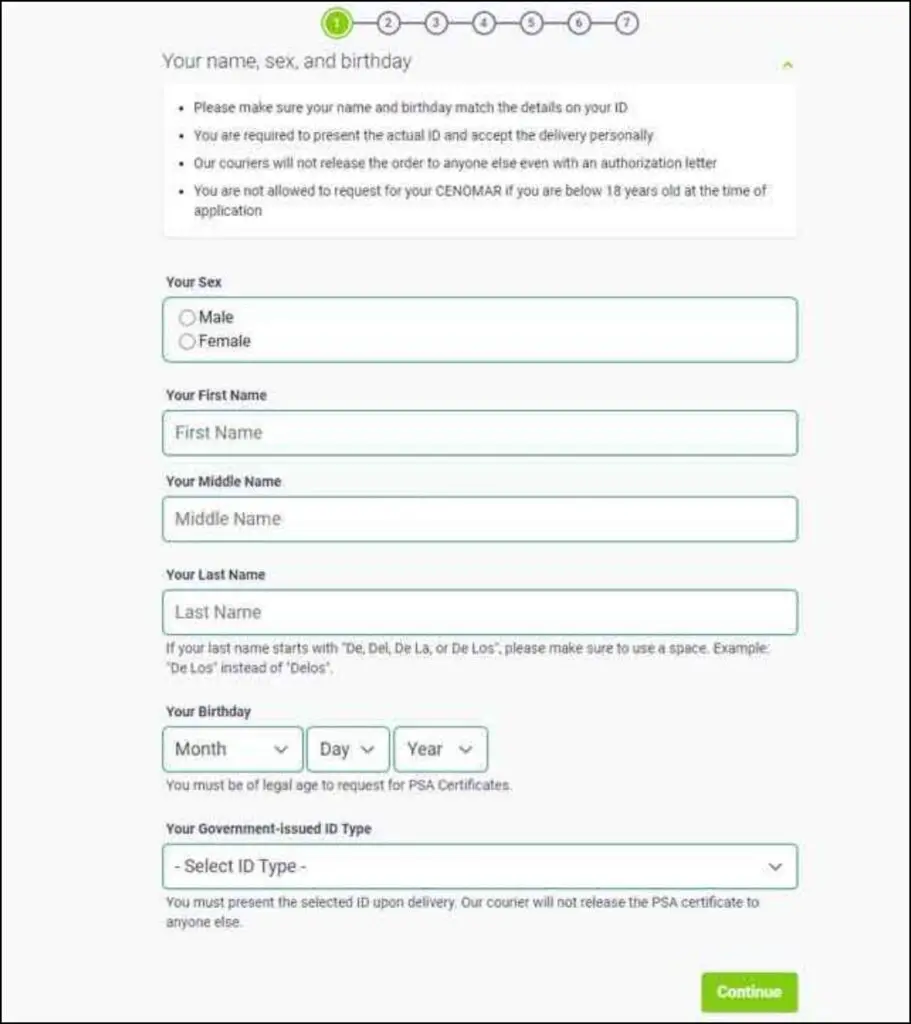The image depicts a gray background webpage with a distinct black border framing the entirety of the content. At the top, there are a series of numbered circles from 1 to 7, with the number 1 highlighted in green, indicating the current step in a process.

Below this, a white text box contains instructions in gray font, asking users to enter their name, sex, and birthday. Following these fields, there is a notice in bold that reads: "Please make sure your name and birthday match the details on your ID. You are required to present the actual ID and accept the delivery personally. Our couriers will not release the order to anyone else even with an authorization letter."

Further details clarify that individuals under 18 years old cannot request their CNOMAR. The form includes fields for "First Name," "Middle Name," and "Last Name," with a special instruction for last names starting with "DEDI," "DELA," or "DELOS" to ensure the format includes a space (e.g., "DE LOS" instead of "DELOS").

The form also requests the user's birthdate broken down into "Month," "Day," and "Year," emphasizing that legal age is required to request PSA certifications. There is a drop-down menu to select the type of government-issued ID, which must be shown upon delivery.

At the bottom of the image, a green button labeled "Continue" is clearly visible, prompting the user to proceed to the next step.